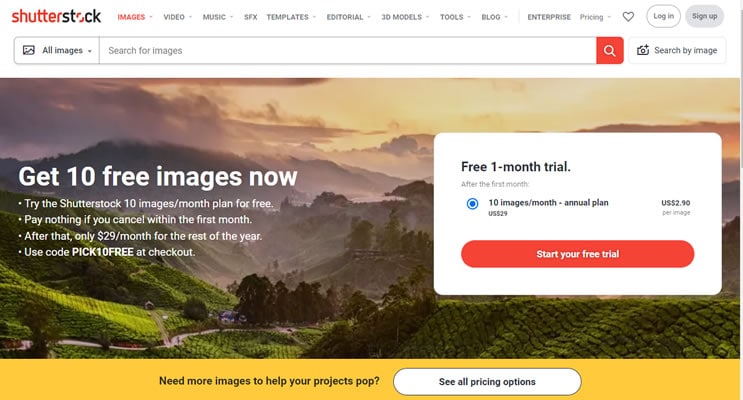The top section of the webpage showcases the Shutterstock logo followed by a navigational menu with options: Images, Video, Music, SFX, Templates, Editorial, 3D Models, Tools, Blog, Enterprise, and Pricing. Adjacent to the menu is a heart icon, a white "Login" button, and a gray "Sign Up" button. Below this, you’ll find a toolbar featuring two search boxes labeled "Search for Images" and "Search by Image." 

Underneath, there is a visually captivating image of mountains terraced with crops, set against a cloudy, purple-hued sky. Accompanying the image is a promotional banner that reads "Get 10 Free Images Now," with four bullet points explaining the offer: 

1. Try the Shutterstock 10 Images/Month Plan for free.
2. Pay nothing if you cancel within the first month.
3. After that, only $29 a month for the rest of the year.
4. Use code PICKONE or PICK10FREE at checkout.

To the right of these details, a prominent button labeled "Start Your Free Trial" encourages users to take advantage of the offer.